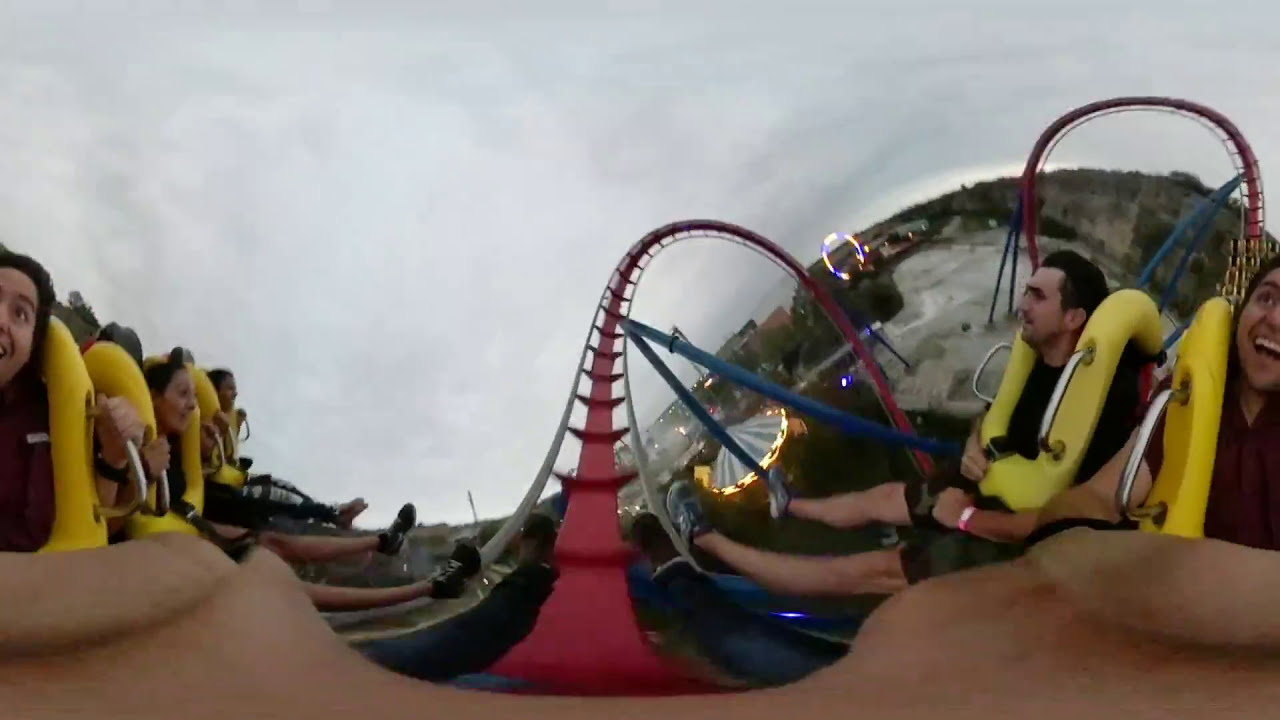In this vibrant and dynamic photograph, people are enjoying an exciting ride on an outdoor roller coaster. The image has been captured with a fisheye lens, giving it a curved, panoramic appearance that merges different sides together. The roller coaster features a striking red track with multiple loopy curves, supported by sturdy blue bars. The ride's seats are equipped with yellow seat belts and cushioning, securing the riders and adding a pop of color to the scene.

Riders, some of whom are laughing, are positioned towards the left and right sides of the image, with their faces visible above their yellow seat restraints. You can even see their hands gripping the metal safety bars and feet sticking straight out in the middle bottom section of the photo. Additionally, part of a hand appears in a kaleidoscope-like effect at the bottom of the frame.

Beneath the roller coaster, the ground is visible, revealing trees, buildings, and the layout of an amusement park adorned with different lights. Above, the sky is primarily overcast with gray clouds, but patches of blue peek through, creating a contrasting backdrop to the thrilling scene below.